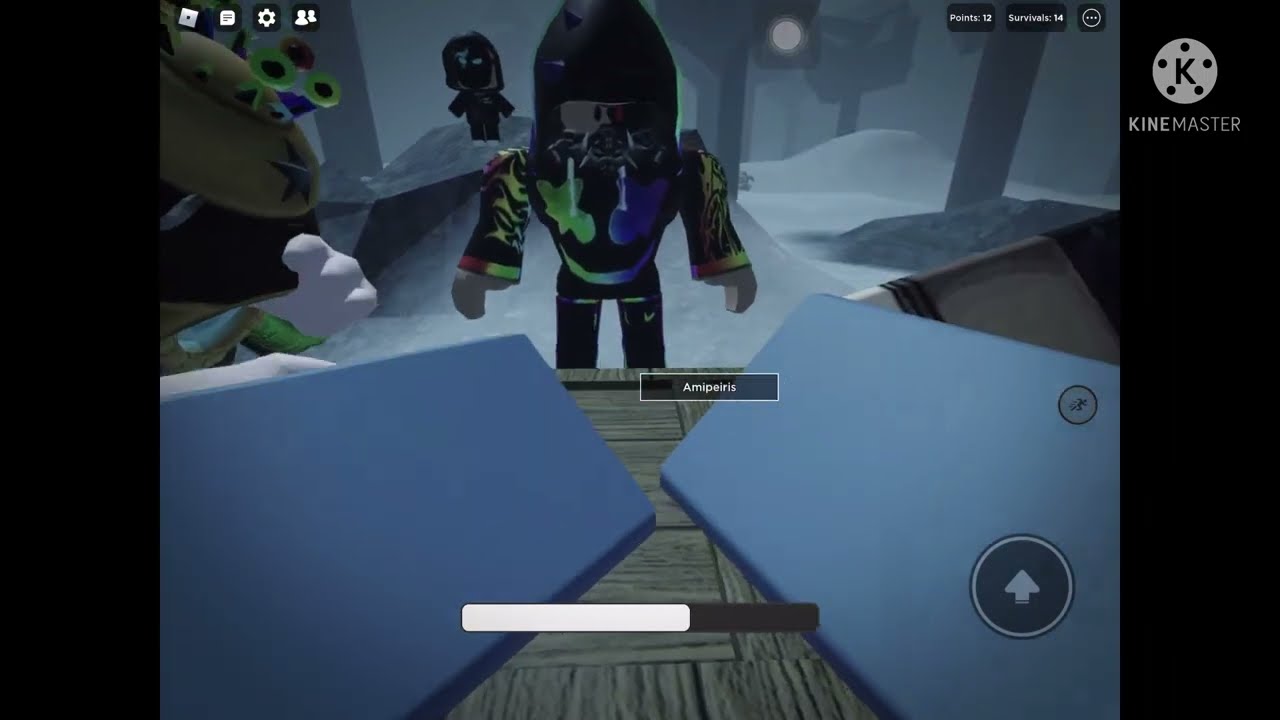In the image, which is a screenshot from a video game, the left and right sides of the screen are bordered in black. At the very top right corner, there is a white circle with a black letter "K" in the center and five black dots outlining the "K," followed by the text "KineMaster." The center of the screen displays the game, which features simple, blocky, almost Lego-like graphics. The background appears to be a misty woodland with snowy hills and trees. 

A central character, clad in a multicolored long-sleeve top (with black, purple, green, and red) and black pants, wears a large black helmet. His helmet's visor reveals two distinctively colored eyes, one purple and one green, with the mouth section showing both colors. His sleeves have yellow fire stripes. There are gray hands extending into the screen, possibly robot arms or junk, and on the right side is a dark gray circle with an upward-pointing arrow.

At the bottom of the screen is a life or energy bar, a long horizontal rectangle filled a little over halfway with white and the rest black. The screen also shows various game menus and icons, such as a home button, a text box speech button, a gearbox for settings, and icons of two people, along with other symbols indicating points and survival stats. Additionally, there's a dark gray small circle button with an icon of a person running. 

In the background, a hooded figure in black stands on a rock, and another small character with a hamburger-shaped head and green Martian eyes appears to the left. Together, these elements contribute to the overall rough and simple aesthetic of the game.